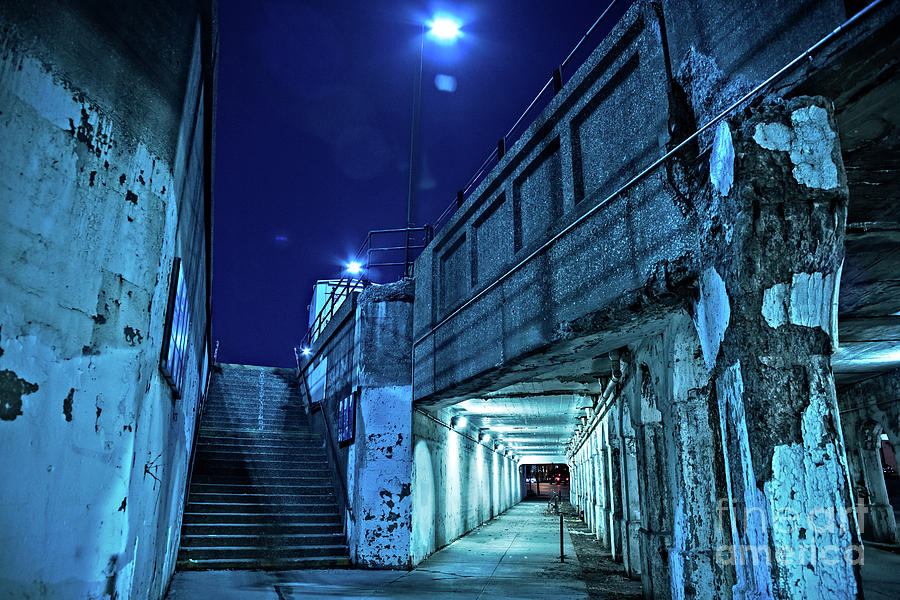Under a clear, dark night sky, this image captures the underside of a street bridge, revealing a pedestrian tunnel illuminated by a series of lights. The tunnel, centered in the picture, stretches into the distance, its aged and worn cement walls showing significant ruin and chipping paint. Ascending from the tunnel, a staircase leads up to the bridge above, where streetlights cast their glow, contributing to the blue tint that seems to permeate the scene. At the bottom right corner of the image, the words "Fine Art America" are faintly visible, adding a subtle watermark to the scene.